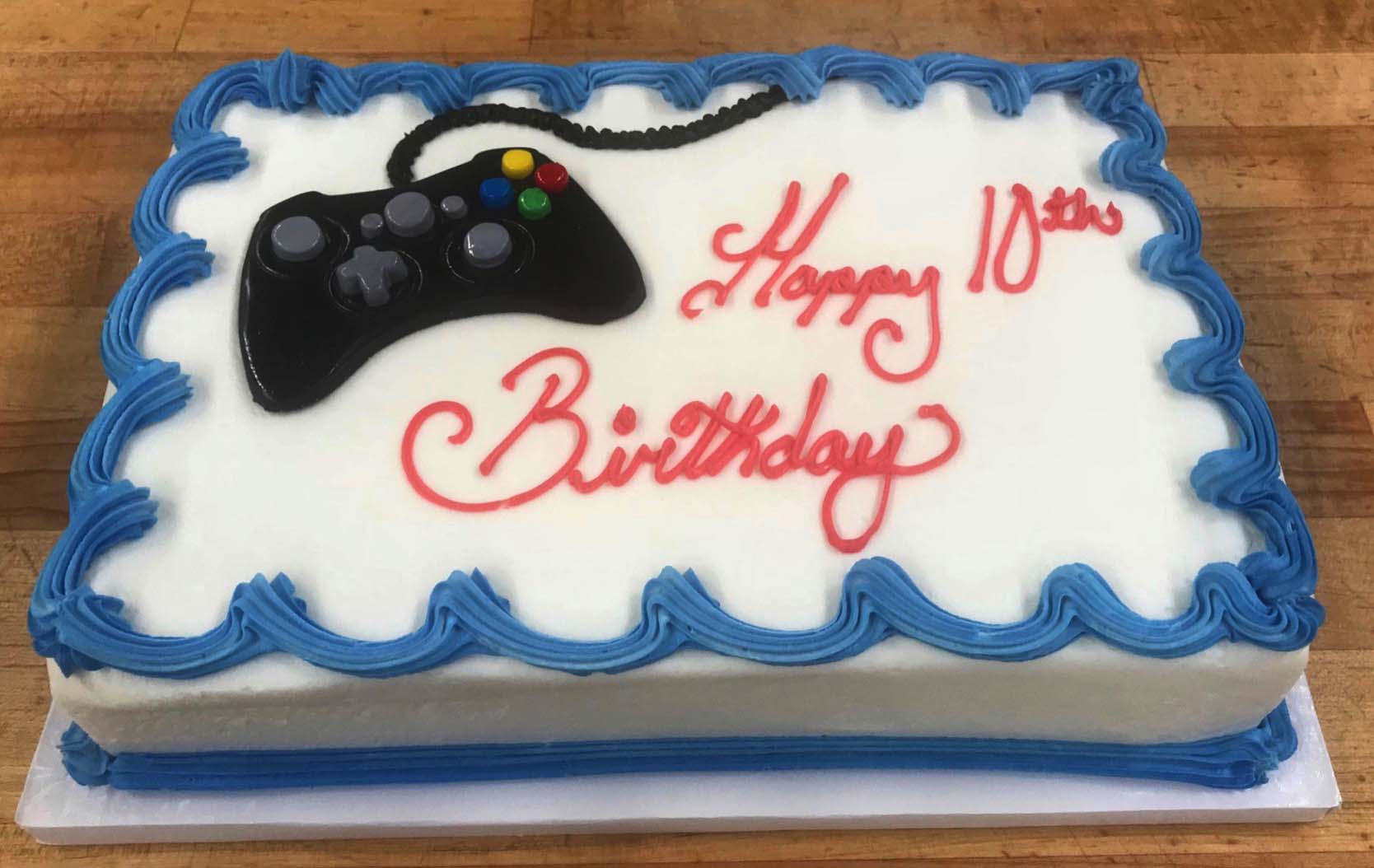The image portrays a rectangular sheet cake adorned with white icing, set on a white serving platter atop a brown wooden table. The cake is decorated with swirly blue trim on both the top and bottom edges. In the center of the cake, slightly off to the right, "Happy 10th Birthday" is written in red script icing. On the upper left side of the cake, there is a lifelike image of a black Nintendo controller. The controller is detailed with gray buttons and colorful buttons arranged in a cross pattern: red to the right, yellow at the top, green at the bottom, and blue to the left. A black cord trails from the controller to the top of the cake, adding to its realistic appearance.